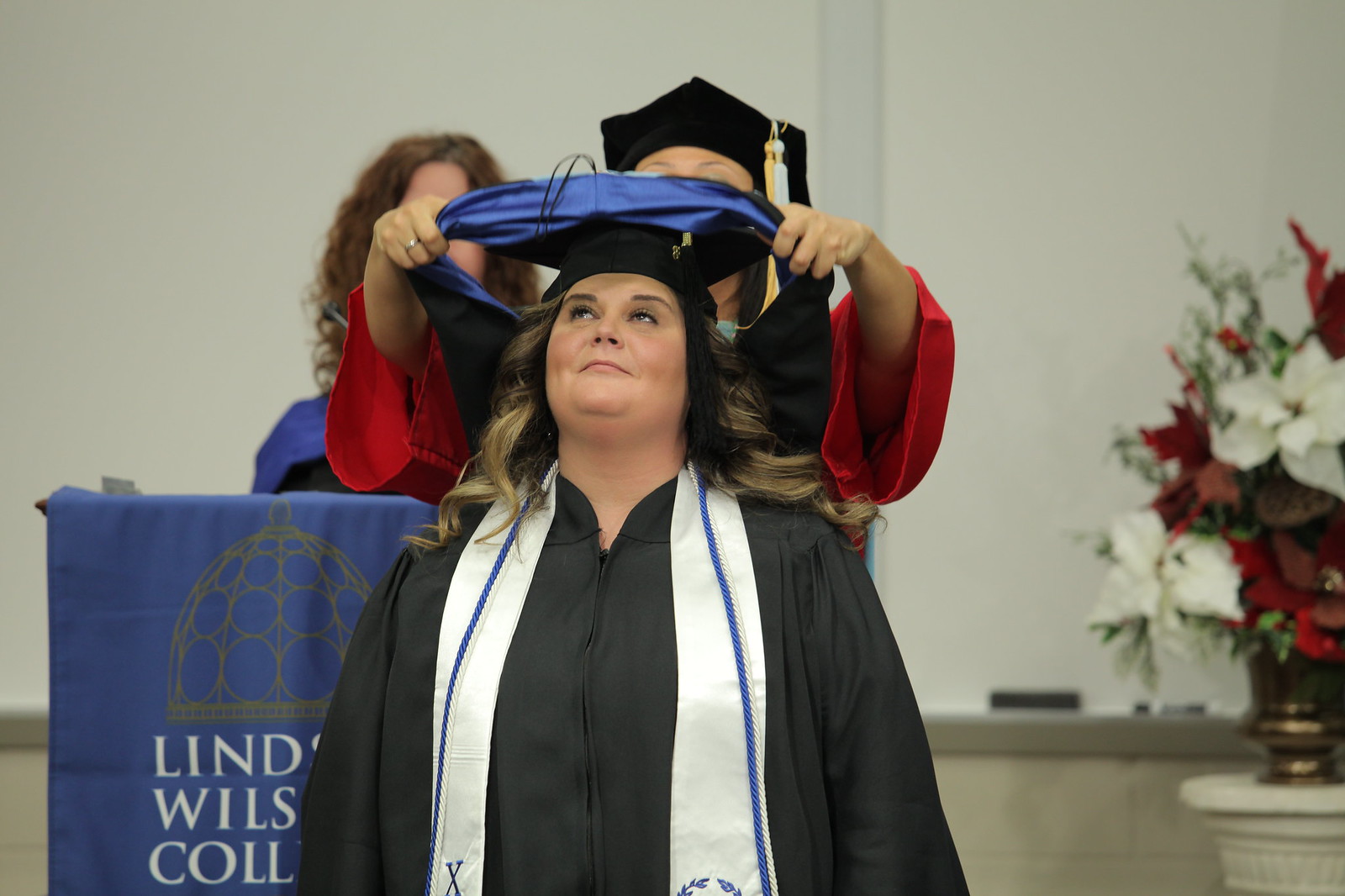The image depicts a graduation ceremony, featuring a prominently positioned woman dressed in a black graduation robe, adorned with a white sash accented by blue stripes, and wearing a graduation cap. She appears to be receiving an award, possibly indicating her status as a valedictorian. Behind her, another individual in a red robe and black hat is placing a blue ribbon around her neck. On the stage, a third person with long curly hair stands behind a podium, which is draped in a blue banner bearing what seems to be the gold logo of Lindsay Wilson College. The background reveals a white wall and a small pedestal holding a bouquet of white and red flowers in a gold vase. The celebratory atmosphere is underscored by these decorative elements, highlighting the significance of the occasion.